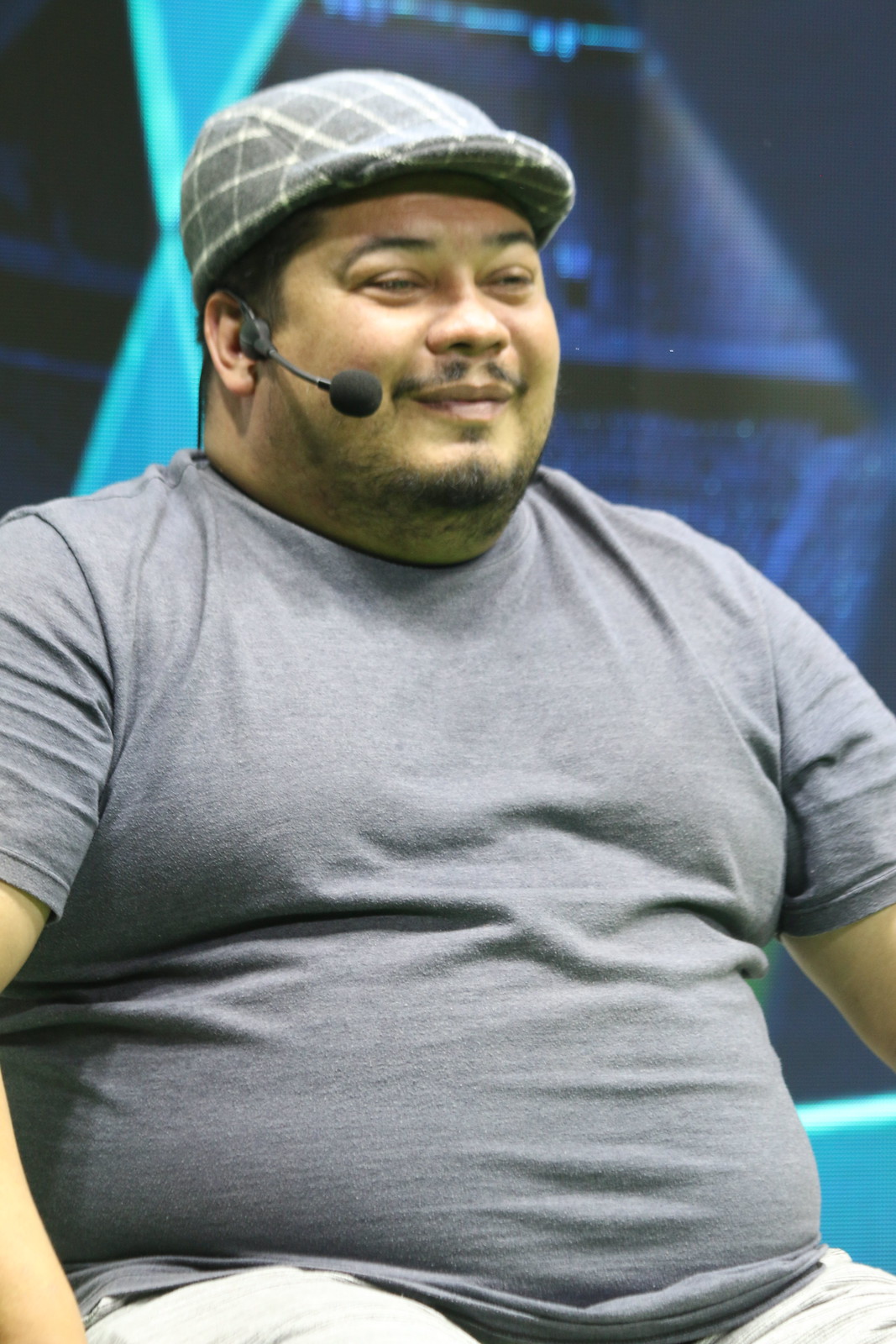The photograph captures a hefty man in his 30s or 40s, sitting down and smiling at something to his right. He wears a gray short-sleeved shirt and white pants, along with a gray cap featuring white stripes. A microphone headset is positioned at his mouth, enhancing the impression that he is engaged in a speaking role, possibly on a stage or podium. His facial hair includes a black mustache and small black stubble. Behind him, the background features a blue wall with light blue geometric designs, adding a modern and visually engaging element to the scene. The photo is in portrait orientation and employs a realistic, representational style.